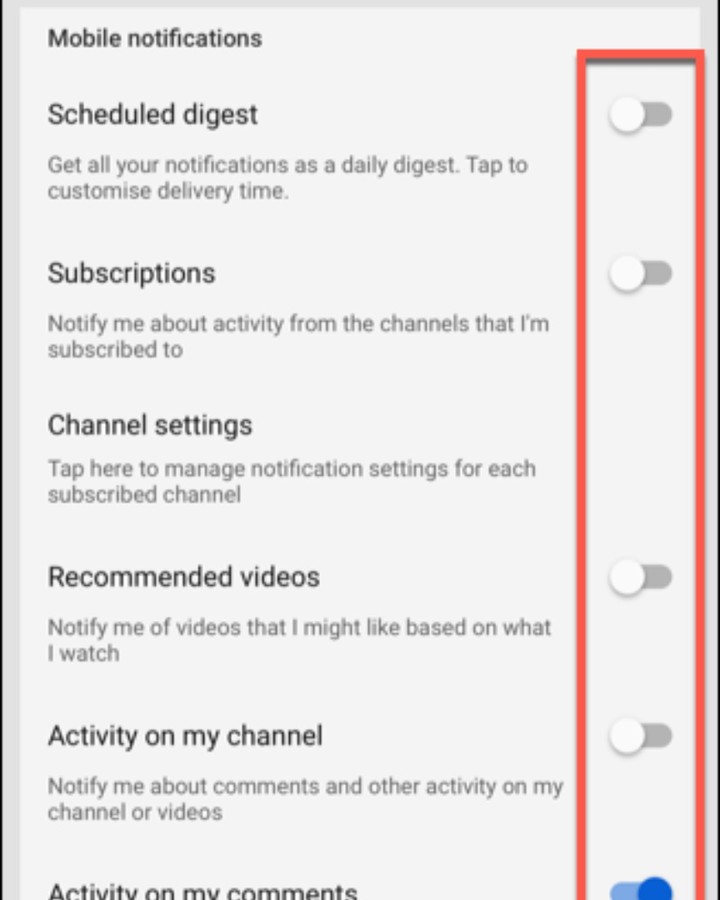This color image showcases a mobile notification settings screen for an unknown app. The header at the top reads "Mobile Notifications" and "Scheduled Digest." Below this, the text explains that users can receive all notifications as a daily digest and can tap to customize the delivery time. 

On the right side, there is a red-bordered section featuring toggle buttons for various notification options:

1. "Scheduled Digest" is turned off.
2. "Subscriptions" is off, which pertains to notifications about activity from subscribed channels.
3. "Channel settings" is off, inviting users to manage notifications for each subscribed channel.
4. "Recommended videos" is off, referring to notifications about videos that might interest the user.
5. "Activity on my channel" is off, for notifications about comments and other activities on the user's channel or videos.
6. "Activity on my comments" is turned on, indicated by a blue toggle button.

The background is white with black text, and there are no photographic elements in this image. The image cuts off just below the "Activity on my comments" section.